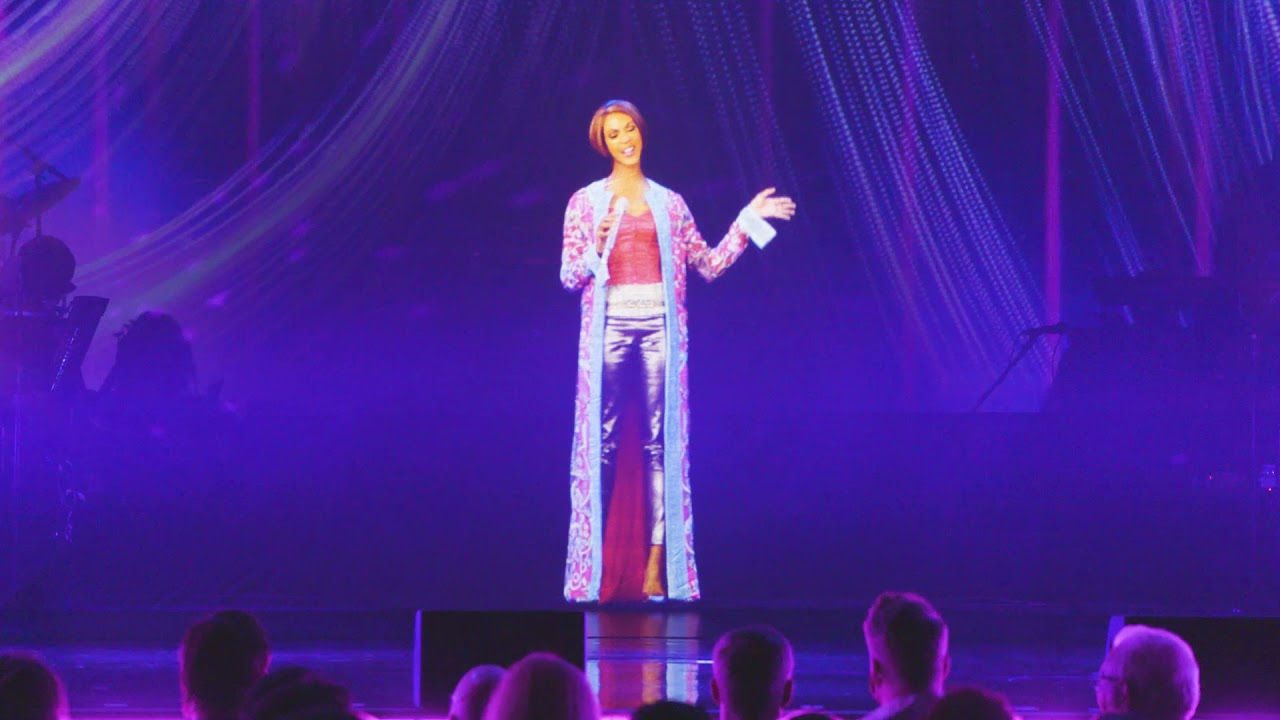The image captures the captivating scene of a hologram concert, featuring a woman standing center stage in a mesmerizing array of purple, blue, and pink lighting. She is clad in a stunning long, multi-colored robe with a pink top and shiny silver pants. The woman, who has short brown hair, appears animated and engaging, holding a microphone in her right hand while her left hand is outstretched, deep in the act of either singing or giving an impassioned presentation. The audience is seen from the back, their heads filling the foreground as they are engrossed in the performance, which includes additional elements like a drum set to the left and a DJ stand to the right. The backdrop is smoky, giving an ethereal atmosphere, enhanced by a curtain of small lights hanging down and casting a glow that makes the hologram look strikingly lifelike. The venue feels intimate and dim, resembling a club, with the shadowy figures and instruments creating an almost abstract and surreal ambience.